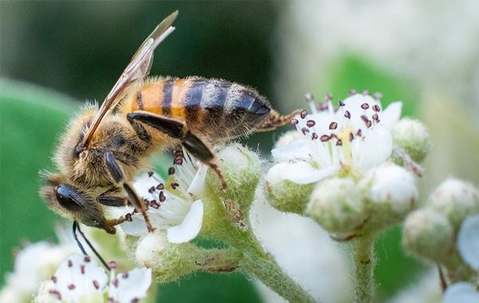In this close-up, vividly colored photograph taken outdoors, a honeybee is meticulously gathering pollen on a cluster of white, cottony flowers speckled with tiny red dots. The bee, positioned with its head nearly upside down in the center of the bloom, has its wings proudly raised and its stinger visible on the right. Its body, adorned with striking gold and brown vertical stripes, glimmers against the textured green stems of the plants, which appear to have fine, fibrous hairs. The background is a blur of greens and whites that blend into a natural, out-of-focus tapestry, enhancing the sharp, detailed foreground where the bee busily collects nectar, looking content as it works.